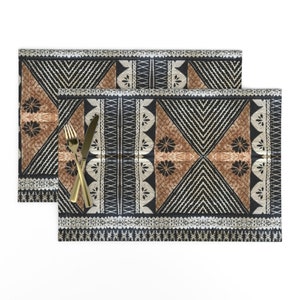This color photograph depicts two intricately designed placemats, one positioned slightly askew atop the other, arranged as if for a product thumbnail. The upper left placement of the top mat showcases a gold fork and knife crossed at the handles for decorative presentation. The geometric design features a distinct southwestern flair, predominantly in black, white, and brown tones. The pattern consists of crisscrossing lines forming layered triangles with two prominent brown triangles adorned with black floral star shapes. These are complemented by white sections with delicate black lace-like lines. Two black bands with white X patterns adorn the top, bottom, and right edges of the placemats, while additional black and white striped triangles and arched patterns enhance the intricate design, all set against a stark white background. This sophisticated pattern, reminiscent of southwestern decor yet modernized for appeal, is typical in regions like Arizona.